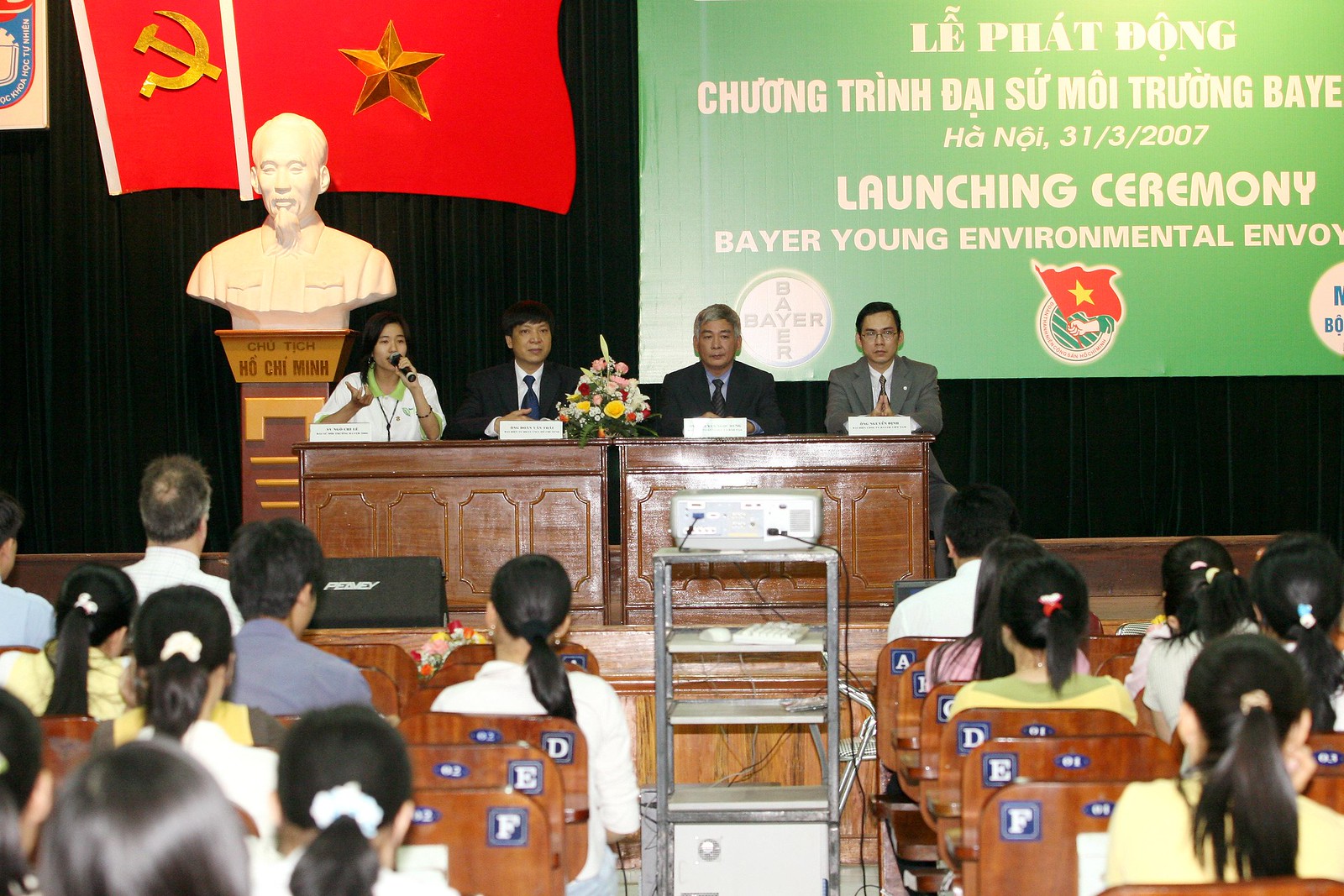The image depicts a formal event taking place in a large auditorium with a sizable audience seated in wooden chairs. Four individuals, comprising three men in suits and a woman in a white polo shirt with green trim, are seated at two brown desks on a stage at the front of the room. The men on the right are dressed in gray and black suits, respectively, and the man next to the woman on the left is also wearing a black suit. A notable backdrop includes a statue of Ho Chi Minh, visible from his shoulders up and white in color, positioned on a mantel-like structure. Behind the stage, two flags are displayed prominently: one featuring a gold star on a red background and another with what appears to be an anvil and axe. A large green banner with white lettering bearing both Vietnamese language and the phrases "Launching Ceremony" and "Be Your Young Environmental Envoy" is also present. The audience comprises individuals of various ages, with some appearing to be young students. The scene suggests a formal presentation, potentially of political or environmental significance, with a projector screen displaying corresponding messages in the auditorium.